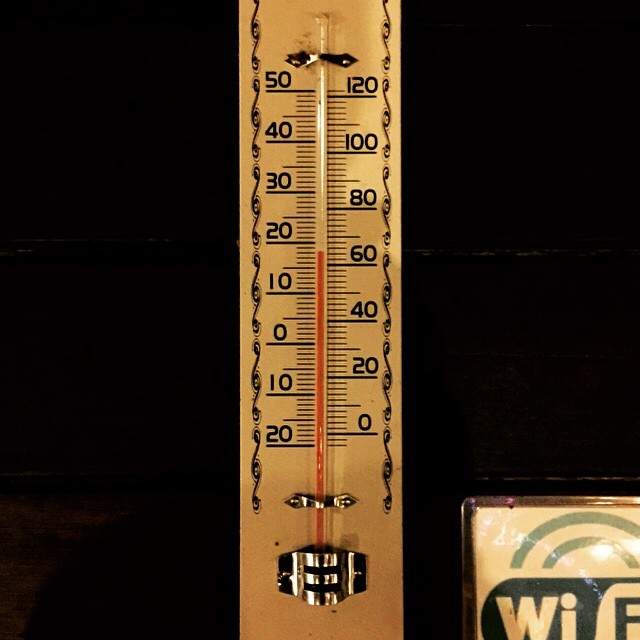The image displays a vintage mercury thermometer set against a black background. The thermometer features a dark brown body with black numerals. A central bar houses a visible red mercury line. The temperature scale on the thermometer ranges from 20 to 50 degrees Celsius and 0 to 100 degrees Fahrenheit. On the bottom right corner, partially cut off, there is a square icon with the word "Wi-Fi" and a green semi-circle above it. The sides of the thermometer are adorned with black, wavy lines, adding an element of intricate detail. The overall composition of the photograph is minimalistic, drawing focus to the unique features of the thermometer.